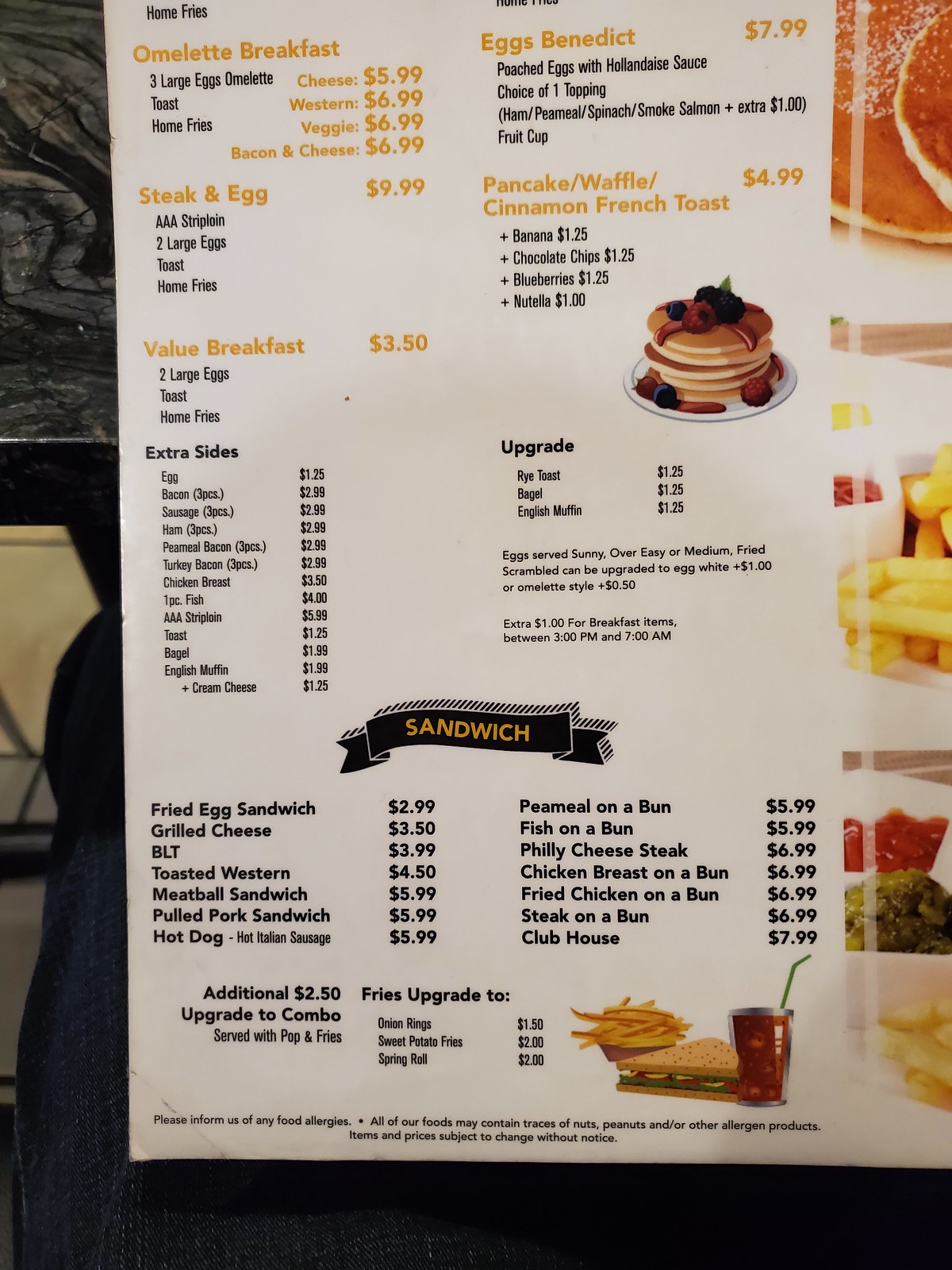The image showcases a laminated restaurant menu set against a white background. To the left, a mosaic-like, abstract design in dark grays and blues, with a black stripe, transitions into a yellow-colored wall. The top-left corner of the background features a chair back. The bottom of the image is black, grounding the menu.

The menu prominently displays breakfast items and includes a notice at the bottom: "Please inform us of any food allergies. All of our foods may contain traces of nuts, peanuts, and/or allergen products. Items and prices subject to change without notice."

On the left side of the menu, several pictures can be seen: a pair of pancakes in the top-right corner, a sunny-side-up egg with a bowl of ketchup and French fries below it, followed by an image of French fries alongside a bowl of greens.

Highlighted in yellow, the major menu categories include:

- **Omelet Breakfast**: Featuring three large egg omelets, toast, home fries, cheese, Western veggie options, and bacon and cheese, with prices provided for each.
- **Steak and Eggs**: Priced at $9.99, with a description of ingredients.
- **Value Breakfast**: Priced at $3.50, listing extra sides available.
- **Eggs Benedict**: Priced at $7.99, also with a description of ingredients.
- **Pancake, Waffle, Cinnamon French Toast**: Priced at $4.99, with available upgrades.

Below the breakfast items, the menu presents a selection of sandwiches:

- **Fried Egg Sandwich, Grilled Cheese, BLT, Toasted Western, Meatball Sandwich, Pulled Pork Sandwich, Hot Dogs, Pea Meal or Piece Meal on a Bun, Fish on a Bun, Philly Cheesesteak, Chicken Breast on a Bun, Fried Chicken on a Bun, Steak on a Bun, Clubhouse**: Various options with an additional fries upgrade.

This detailed caption provides a thorough description of the menu's content and setting, highlighting the main categories and items available for breakfast.